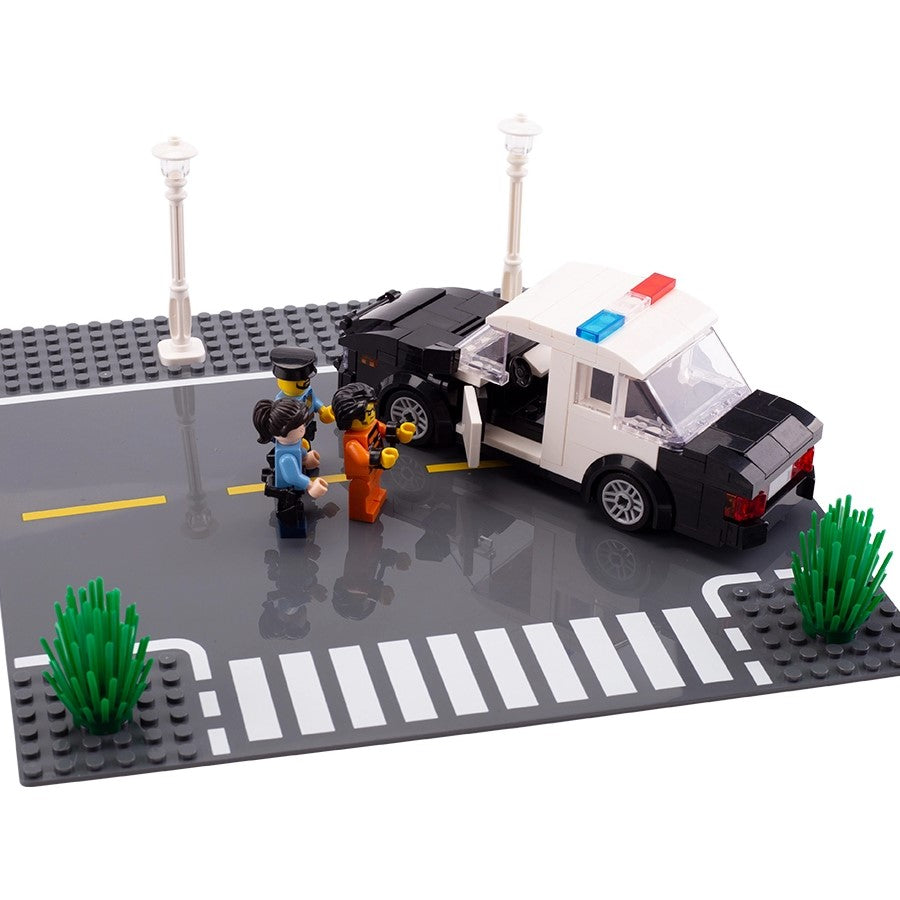The photograph depicts a detailed Lego scene featuring a police operation on a Lego road. At the center is a black and white police car, distinguished by its open door and a red, white, and blue siren on top. The scene shows two Lego police officers, one male with a hat and one female, both dressed in blue police uniforms, escorting a handcuffed Lego criminal in a bright orange jumpsuit. The criminal, who has black hair and an angry expression, is being led into the open door of the police car. The Lego road showcases a yellow dividing line, a crosswalk, and is flanked by two green bushes and two street lamps. This intricate setup vividly portrays the police officers managing the arrest as part of their duty.